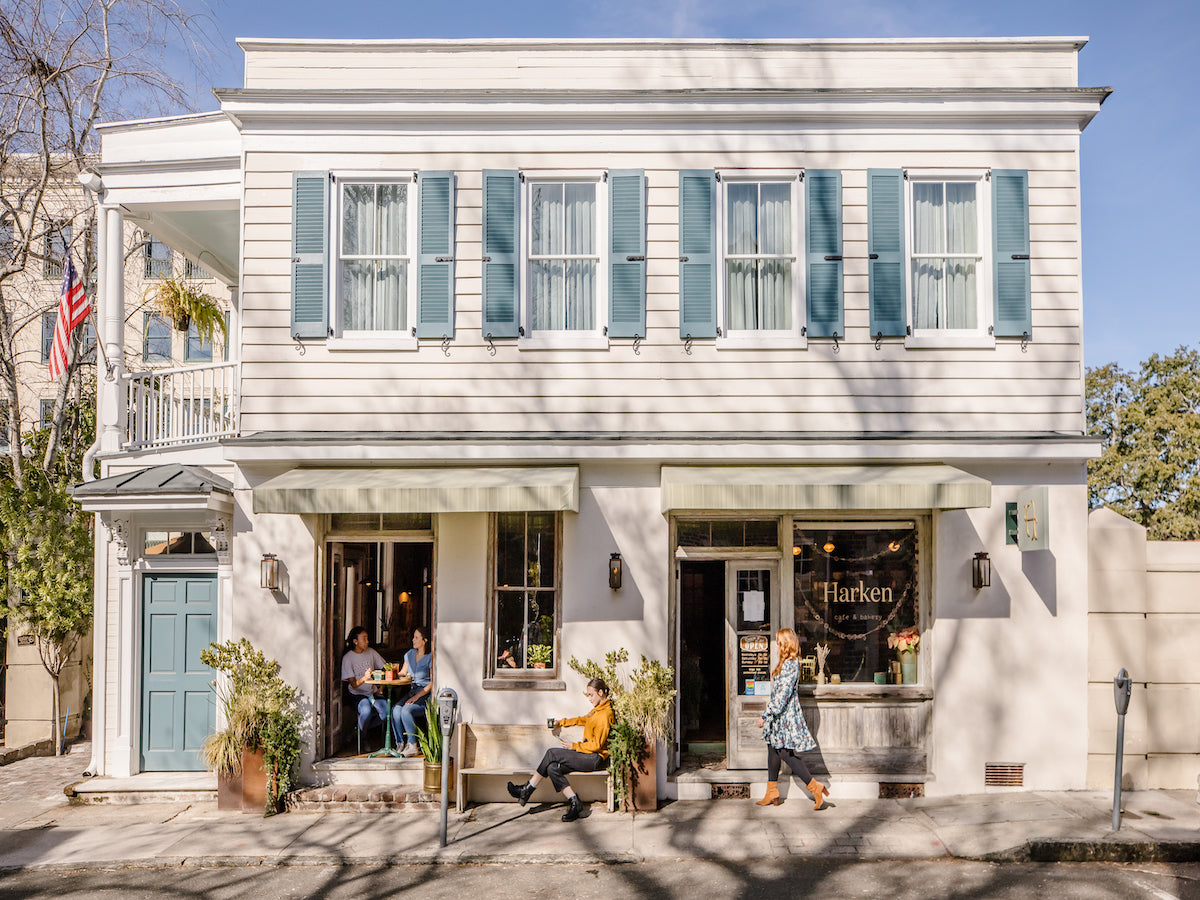The image depicts a small, inviting building set against a clear blue sky with scattered, light clouds suggesting a sunny day. On the bottom right and left edges of the image, lush green trees frame the scene, adding a touch of nature to the urban setting. The predominantly white building features white-framed windows and a distinctive bluish design element, including a matching blue door that highlights its charming façade.

The building, possibly a cozy restaurant or café, bears the name "Harkin" prominently displayed on both the door and window. Near the entrance, a lone individual sits leisurely on a beige bench, holding a black mug, perhaps enjoying a warm beverage and the pleasant weather. Peeking through another entrance, two people can be observed sitting at a table inside, suggesting a welcoming interior. Additionally, a person is captured in motion, walking towards the door, seemingly about to enter the establishment. The scene altogether conveys a sense of tranquility and community activity.